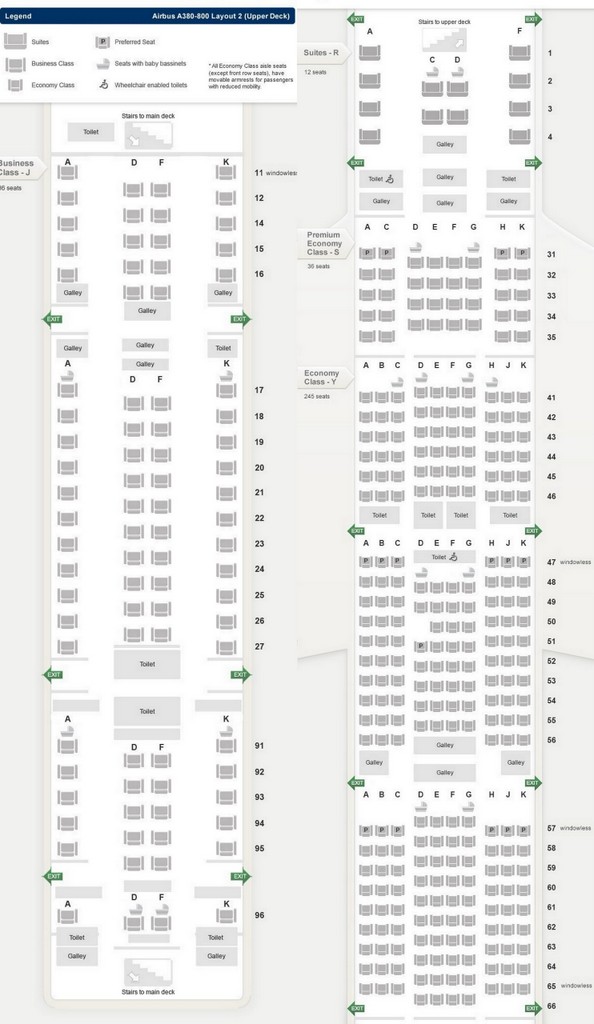This image presents a detailed seating layout for an Airbus A380-800 aircraft, specifically highlighting the upper deck configuration, labeled as "Layout 2." In the upper left corner, a blue bar features the title "Legend," aiding in the interpretation of the seating map.

The upper deck layout categorizes seats into different classes and sections. Business class is depicted with gray seat symbols and is divided into several sections:
- The A section is located on the far left.
- The D and F sections are centered in the middle.
- The K section is on the far right.

Adjacent to the business class sections, the image illustrates the arrangement of suites and preferred class seats. Moving towards the rear, the image transitions to show economy class seating, alongside additional suite areas. The seat numbering extends to at least 96, indicating a substantial passenger capacity.

On the left side of the image, the layout predominantly showcases business class seats, while the right side presents a varied mix of business class, economy, and suite accommodations. This comprehensive depiction provides viewers with a clear understanding of the aircraft's upper deck seating configuration, helping to clarify different seating options and class distinctions within the Airbus A380-800.